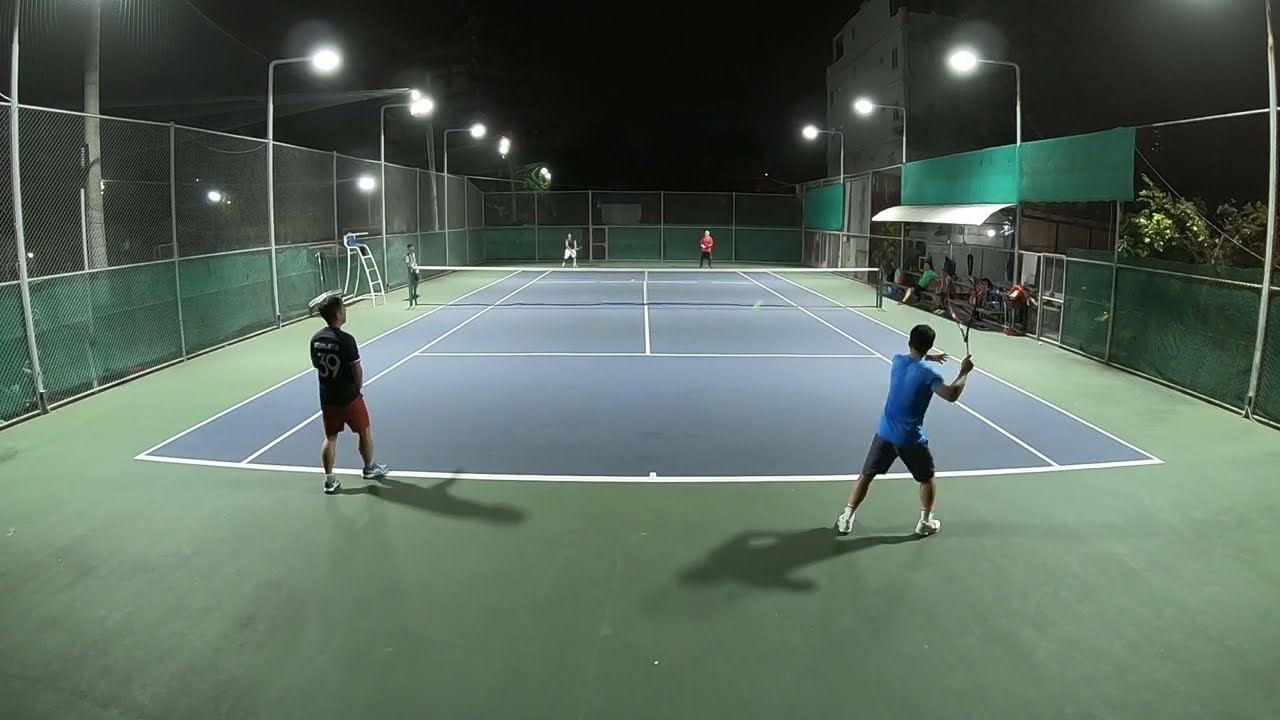The image shows a well-lit outdoor tennis court at night, with distinctive blue and green hard court surfaces marked by white lines. A doubles match is in progress, with two players on each side of the net. The player in the foreground, wearing a blue shirt, is poised to swing his racket upwards, while his teammate in a black shirt with the number 39 stands to his left. The opposing team, clad in red and black shirts, can be seen in the distance. A large chain-link fence with green panels encloses the court. Spectators are scattered around the court, sitting and standing, with some seated under a white overhang near the right side. The court is surrounded by illuminating lights and nearby buildings, enhancing the lively atmosphere of the nighttime tennis match.